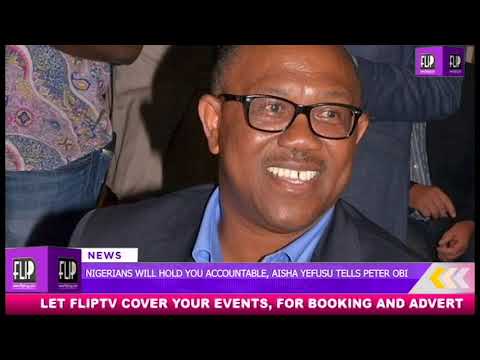The screenshot depicts a TV broadcast featuring an African-American man with a bald head and black plastic-framed glasses. He is smiling, revealing a gap in his teeth, and dressed in a gray suit jacket over a light blue collared shirt. The man is positioned slightly off to the right side of the screen. The TV image is bordered by a plain black header and footer. In the background, partially visible people are discernible, including individuals in a multicolored pink, blue, and yellow shirt, and others wearing gray suits.

A purple banner spans the bottom of the screen with white text that reads: "Flip News, Nigerians will hold you accountable. Aisha Yefusu tells Peter Obi." Below this, against a red background with white text, it says: "Let Flip TV cover your events for booking and advert." The upper right-hand corner displays a purple cube with white and black text reading "Flip."